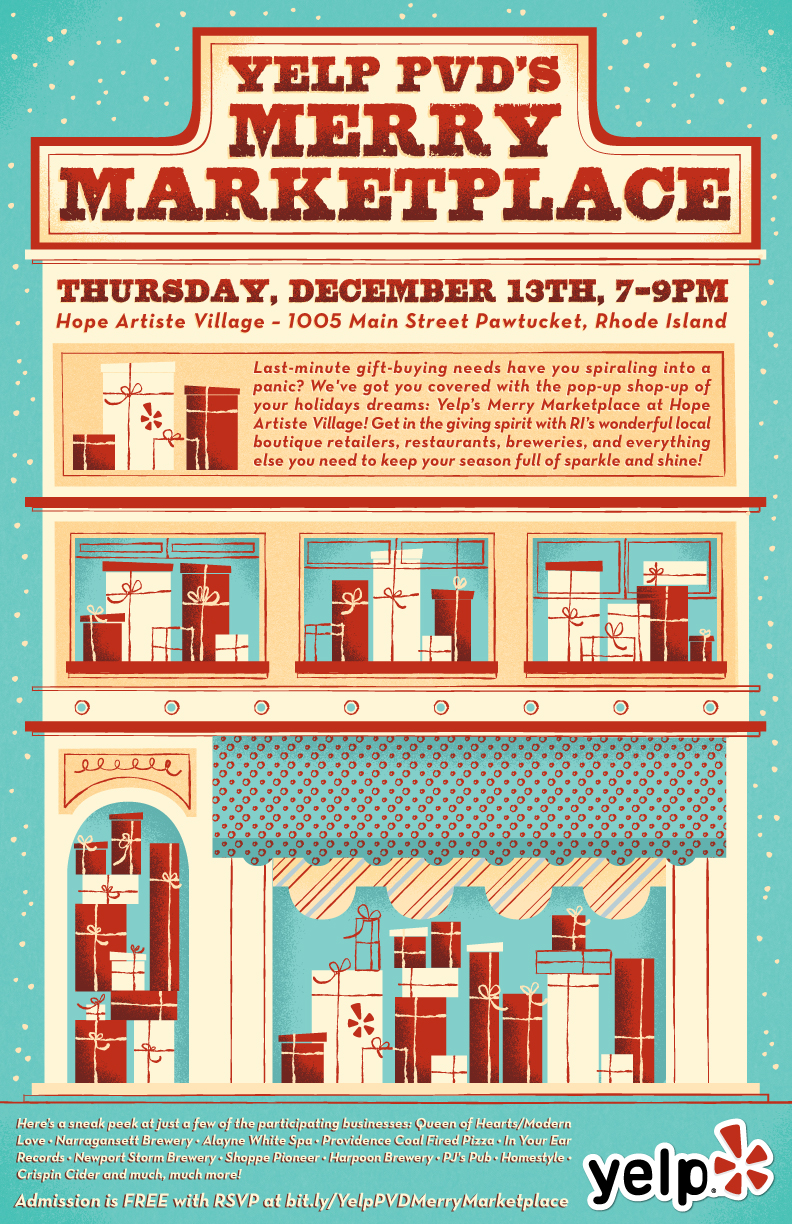This detailed poster created by Yelp advertises "Yelp PVD's Merry Marketplace," set to be held on Thursday, December 13th, from 7 to 9 p.m. at Hope Artiste Village, located at 1005 Main Street, Pawtucket, Rhode Island. The design features a prominent three-story storefront illustration, taking up a significant portion of the image. The first floor showcases an inviting awning in blue and red checks, under which several neatly wrapped gift boxes are displayed. The second floor has windows adorned with additional presents, adding to the festive atmosphere, all set against a light blue background accented with yellow elements. Text details dominate the upper part of the poster, with a mix of red and white fonts on a blue overlay. 

The informational text includes a whimsical description aimed at alleviating last-minute gift-buying stress, promising visitors a delightful pop-up shop experience. The event features various local boutique retailers, restaurants, breweries, and other vendors, highlighting the Rhode Island community spirit. Additional information specifies a sneak peek of participating businesses such as Queen of Hearts Modern Love, Narangasett Brewery, Elaine White Spa, and more, denoted in white text near the bottom of the poster. The bottom right corner features the Yelp logo in black to authenticate the festive advertisement, encouraging viewers to RSVP for free admission via a provided link.